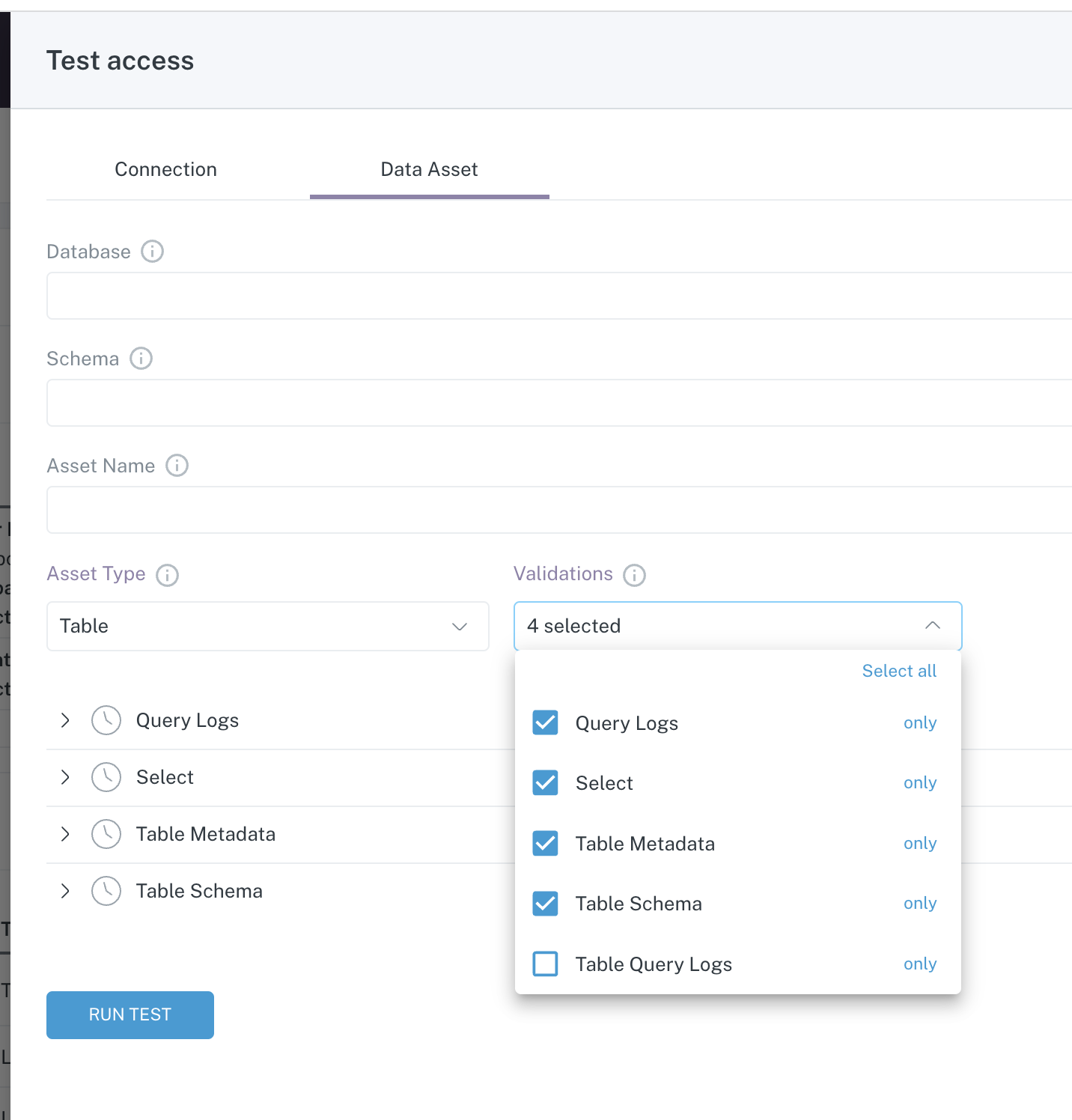A user interface screen displaying test access settings is shown. Centered at the top, in a long gray rectangle, is the heading "Test Access" in black letters. Down the left side of the screen runs a long black vertical bar, potentially part of the software's UI framework. The screen is divided into two main sections: "Connection" and "Data Asset."

The "Data Asset" section is highlighted with an underline, making it the focus. Below this header, there are several fields, each with an accompanying information icon (an 'i' within a circle). These fields include:

1. **Database**: A long text box follows, intended for database input.
2. **Schema**: Another long text box intended for schema input.
3. **Asset Name**: A text box designated for entering the asset's name.
4. **Asset Type**: A dropdown menu with "Table" currently selected. The "Asset Type" field is adjacent to a "Validations" section.

The "Validations" section includes options with checkboxes. The available options are:
- Query Log
- Select
- Table Metadata
- Table Schema

Four options—Query Log, Select, Table Metadata, and Table Schema—are checked. This selection is indicated above by the label "4 selected." A "Select All" option, highlighted in blue, allows for all checkboxes to be selected simultaneously. Each option has an individual "Only" checkbox next to it.

Below these options, a series of lines with greater-than signs (>) and clock icons represent the various validation types. Each line is labeled with one of the selected validation options:
- Query Logs
- Select
- Table Metadata
- Table Schema

At the bottom of the section is a blue button with white text labeled "Run Test," which initiates the testing process.

The fields for entering the database, schema, and asset name are currently blank, awaiting user input. The overall setup appears to be for configuring test access to a database, where the user defines database parameters, validates various data attributes, and ultimately runs a test through the provided interface.